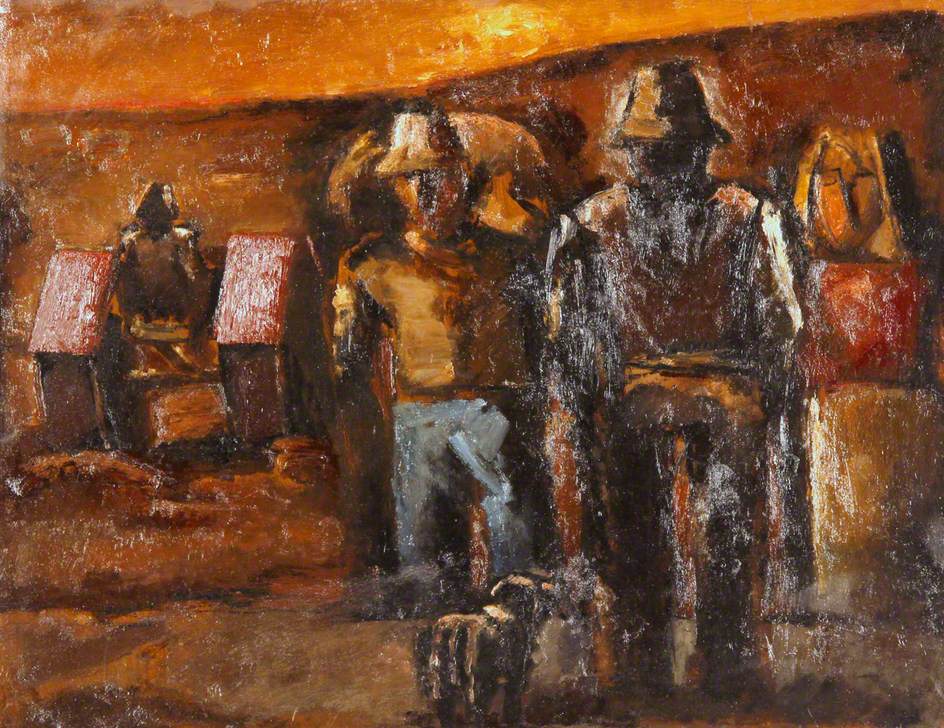The image depicts a detailed painting, horizontally aligned and primarily using shades of brown, dark orange, and intermittent hints of yellow and blue. It portrays a somewhat blurred representation of three figures set against what appears to be a brown-paneled background, which could be a wall or some weathered wooden structures. 

In the leftmost part and center, one figure, wearing a hat and standing between two wooden pillars, is vividly depicted with an upper body and perhaps part of a leg visible. Moving towards the center, two larger figures are present. Both are adorned in hats and sporting attire reminiscent of cowboy clothing. The one on the left is detailed with a brown shirt and gray pants, while the other figure's clothing is less distinct, shrouded in dark hues, perhaps black, and partially obscured by white streaks.

Further right, the artwork subtly depicts various blocks stacked, adding to the composition's depth. There's a possible suggestion of a man in the distance, characterized by a hood and accompanied by a cart, perhaps indicating some form of labor. Flanking this figure are reddish structures, potentially denoting either origins of activity or destinations within this ambiguous yet evocative scene. The figures' faces are indistinct, contributing to the painting's mysterious and atmospheric quality.